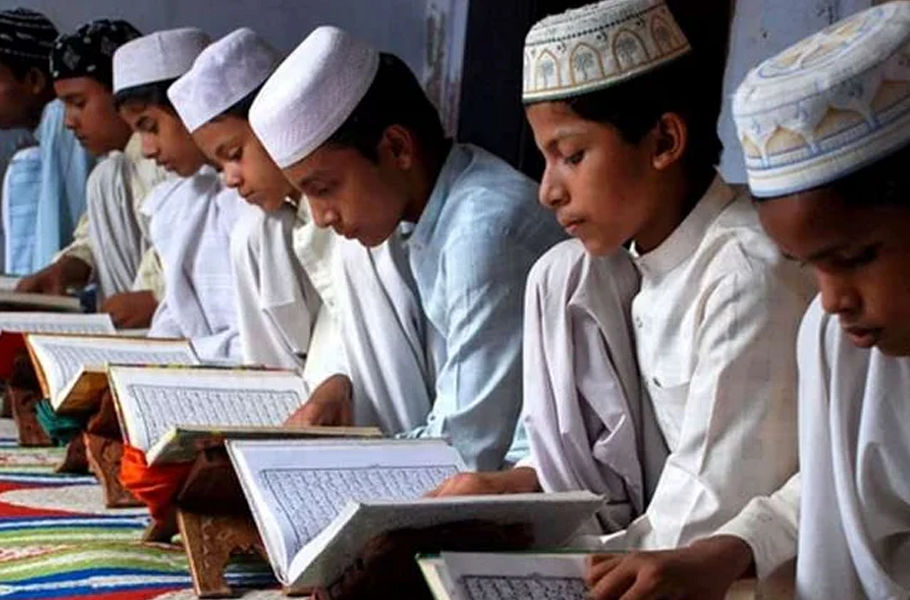The photograph features six young boys, likely between the ages of 10 and 15, who appear to be from a Muslim country. They are seated in a row on the floor, each with their legs crossed on a vividly colored rug that includes primary hues such as greens, reds, yellows, and blues. The boys, who are dark-skinned, are dressed in traditional knee-length garments, similar to those worn by men in India, with some wearing blue and others white. Each boy is also wearing a small hat, which are either plain white or have a subtle print. They are all intently focused on the books in front of them, which are placed on wooden stands. The books contain text that seems to be in a different language, suggesting they could be religious texts. The boys appear to be engaged in religious study or prayer.